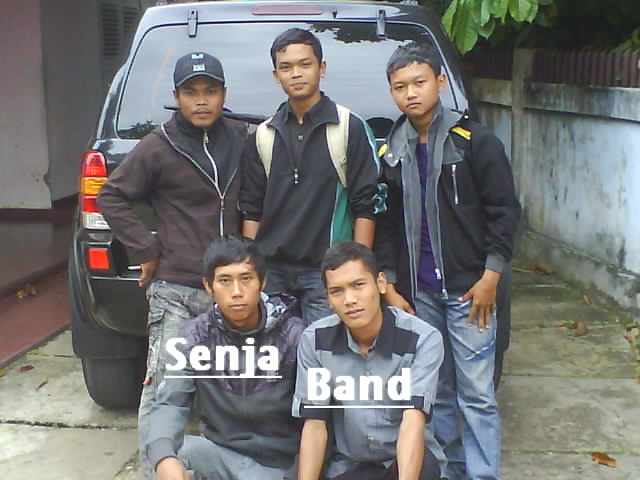In this image, five young Asian men, presumably members of the Sinja band, pose confidently in front of a black SUV. Three of them stand behind the vehicle, while the other two kneel on the concrete ground in front. The central figure, believed to be the singer, exudes a noticeable air of arrogance. The group is dressed mostly in jackets, with one member wearing a t-shirt and another sporting a baseball cap. They are positioned in a nondescript setting, marked by a cement area with visible cracks filled with moss and scattered dead leaves. To the right, a concrete wall topped with spikes frames the scene, while further to the left, a white building wall with a red-painted sidewalk is visible, adding a gritty urban backdrop to their photo.